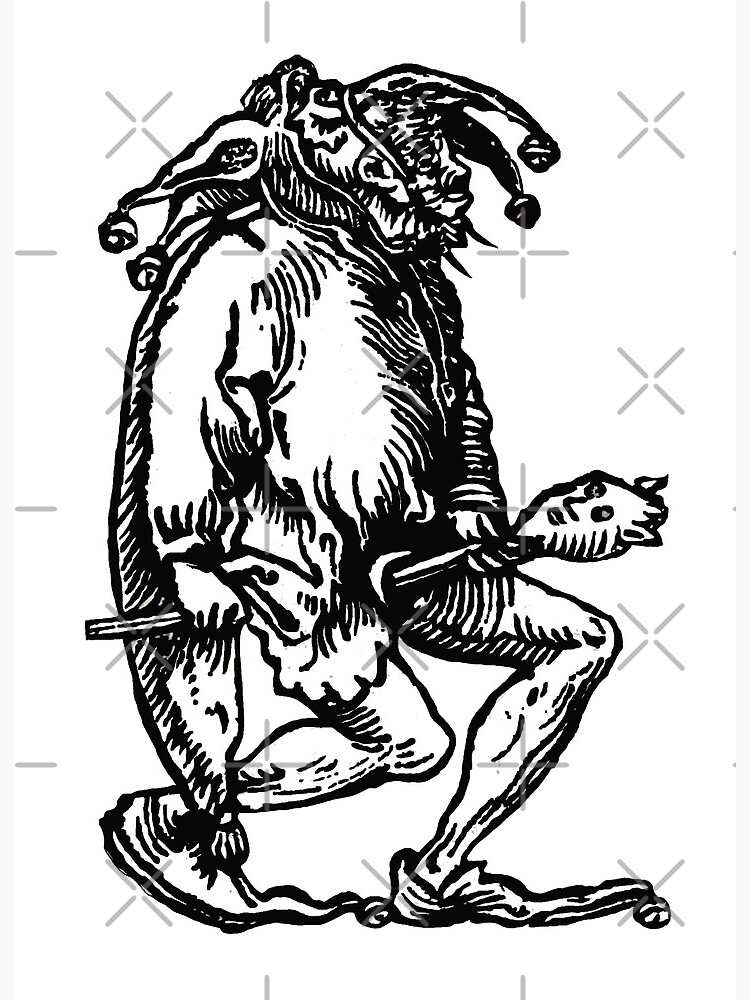The image portrays a detailed black-and-white drawing resembling a character from a medieval comic book. The figure can be best described as a surly, large creature resembling a jester or Joker, characterized by a multi-tiered, elaborate hat adorned with four bells. This jester hat, with its long, pointed ends, extends down almost to his legs. The creature’s face is distorted, giving it a tired and broken-down appearance, adding to its aged look. He is holding a scepter adorned with a head that has eyes, a nose, a mouth, and possibly ears, suggesting a devil or animal-like face. His attire includes shorts and notably wide shoes with long pointed toes accompanied by bells. The entire image is marked with X's, plus marks, and grey watermark lines on all sides, preventing unauthorized copying.